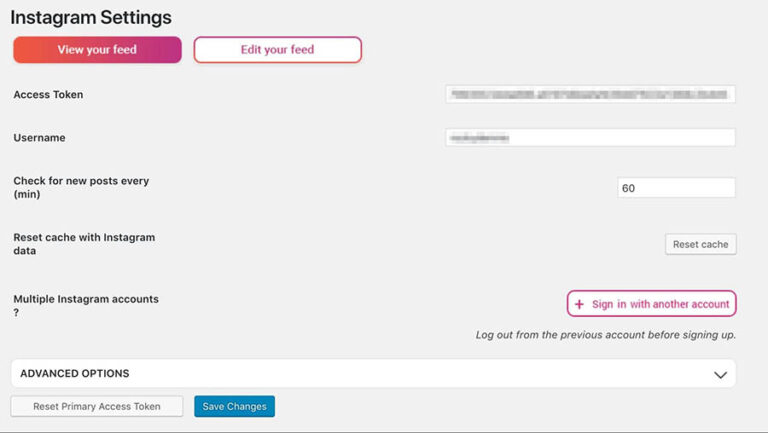The image captures a user interface screen for Instagram settings. At the top left corner, bold black text clearly states "Instagram Settings." Directly below, a red bar displays the option "View Your Feed," followed by a neighboring white bar enclosed in red that reads "Edit Your Feed" in red text. The layout is straightforward and easy to follow.

Further down, in smaller bold black text, the label "Access Token" appears. To the right of this label is a white input area, which has been blurred out, potentially obscuring sensitive information. A substantial gap follows before the "Username" field, also located on the right side and similarly blurred for privacy. 

Below this, there are several options related to post management and cache settings, including "Check for new posts every," with a default value of "60 minutes," and "Reset cache with Instagram data." Additionally, there's a prompt asking "Multiple Instagram accounts?" with an invitation to "Sign in with another account." The screen concludes with "Advanced Options" at the bottom, indicating additional customizable settings for power users.